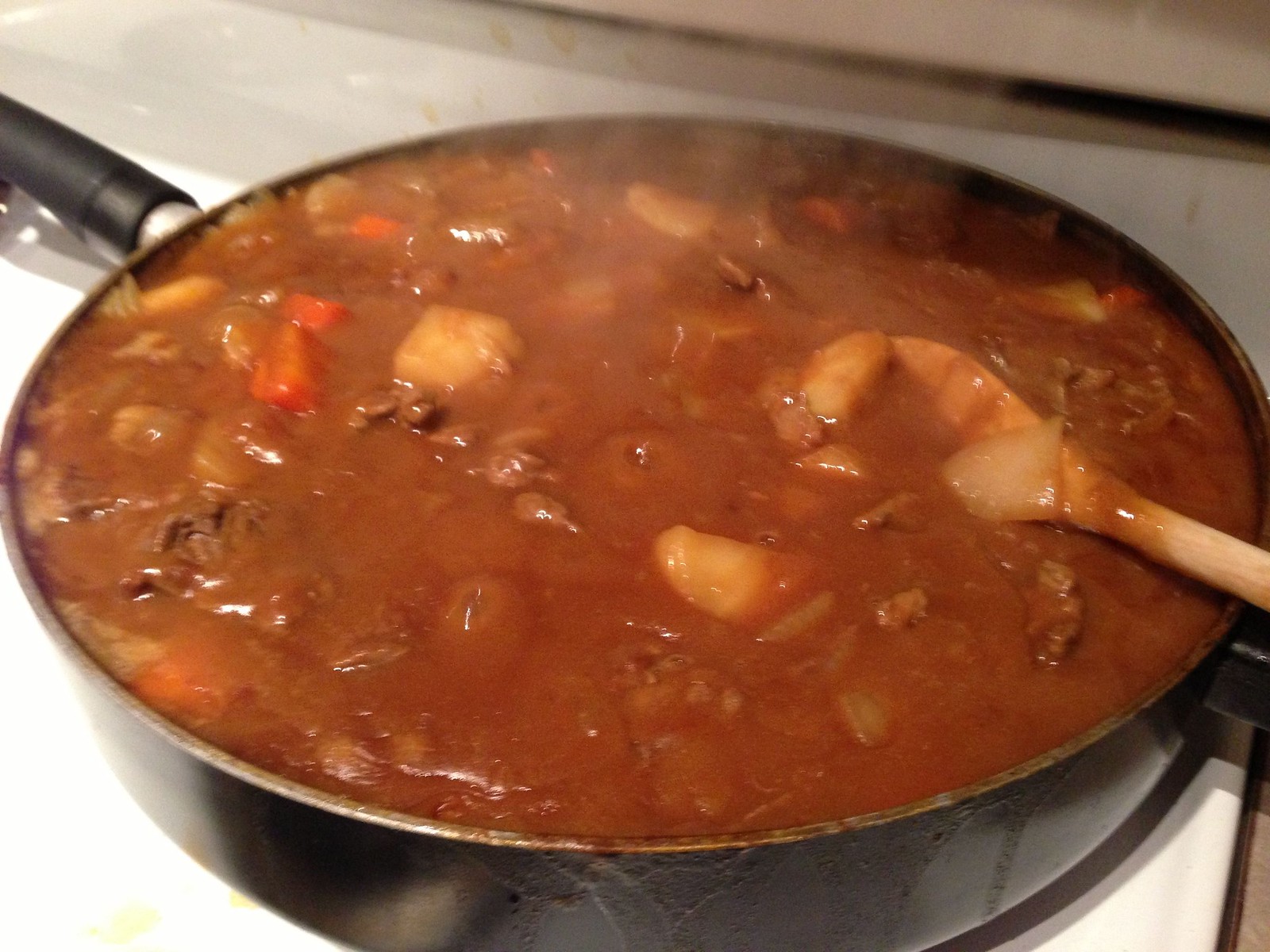The photograph captures a detailed, extreme close-up of an almost overflowing black saucepan situated on a slightly dirty, white stove top. This shiny metal stove surface gleams, accentuating the vivid scene. The main focus is the bubbling, reddish-brown stew simmering vigorously inside the pot, sending wisps of steam into the air. The delicious stew is richly textured with visible chunks of beef, carrots, potatoes, and onions intermixed, creating an appetizing visual. A smooth wooden mixing spoon, partially visible at the edge of the image, is inserted in the pot, revealing bits of potato and onion clinging to it. The black saucepan features a stainless top and sturdy black handles. The scene captures the essence of cooking in motion, with the steaming stew ready to be enjoyed.